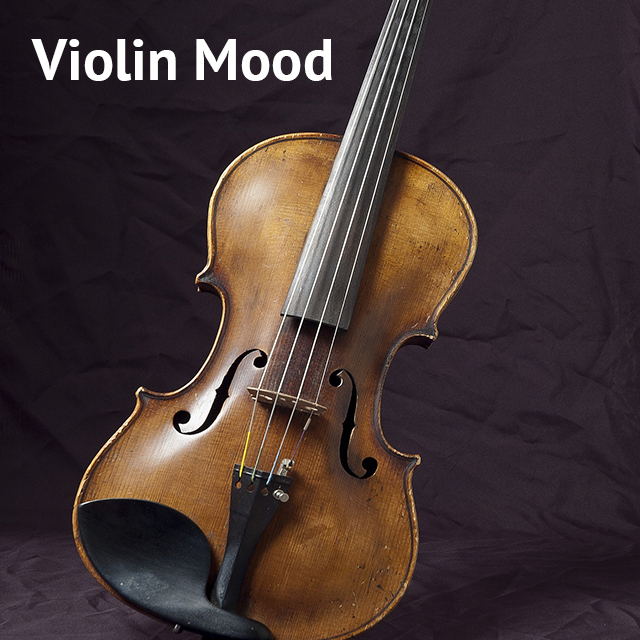This is a studio photograph of an old wooden violin placed at a diagonal angle against a wrinkled dark purple or charcoal-colored fabric backdrop. The violin, featuring a body of medium to dark brown wood with visible chips and darker stained spots, is oriented so that its bottom is near the lower-left corner, and its top extends toward the upper-right corner of the image. Prominently displayed in the upper left-hand corner are the words "Violin Mood," written in capitalized white letters. The violin itself is detailed with several black components, including the chin rest, bridge, and a rounded feature at the bottom. There are two F-shaped sound holes and four vertically aligned silver strings that run from the base, over the black neck, and out of the frame at the top. Light reflections highlight the curves and textures of the instrument, emphasizing its aged character.